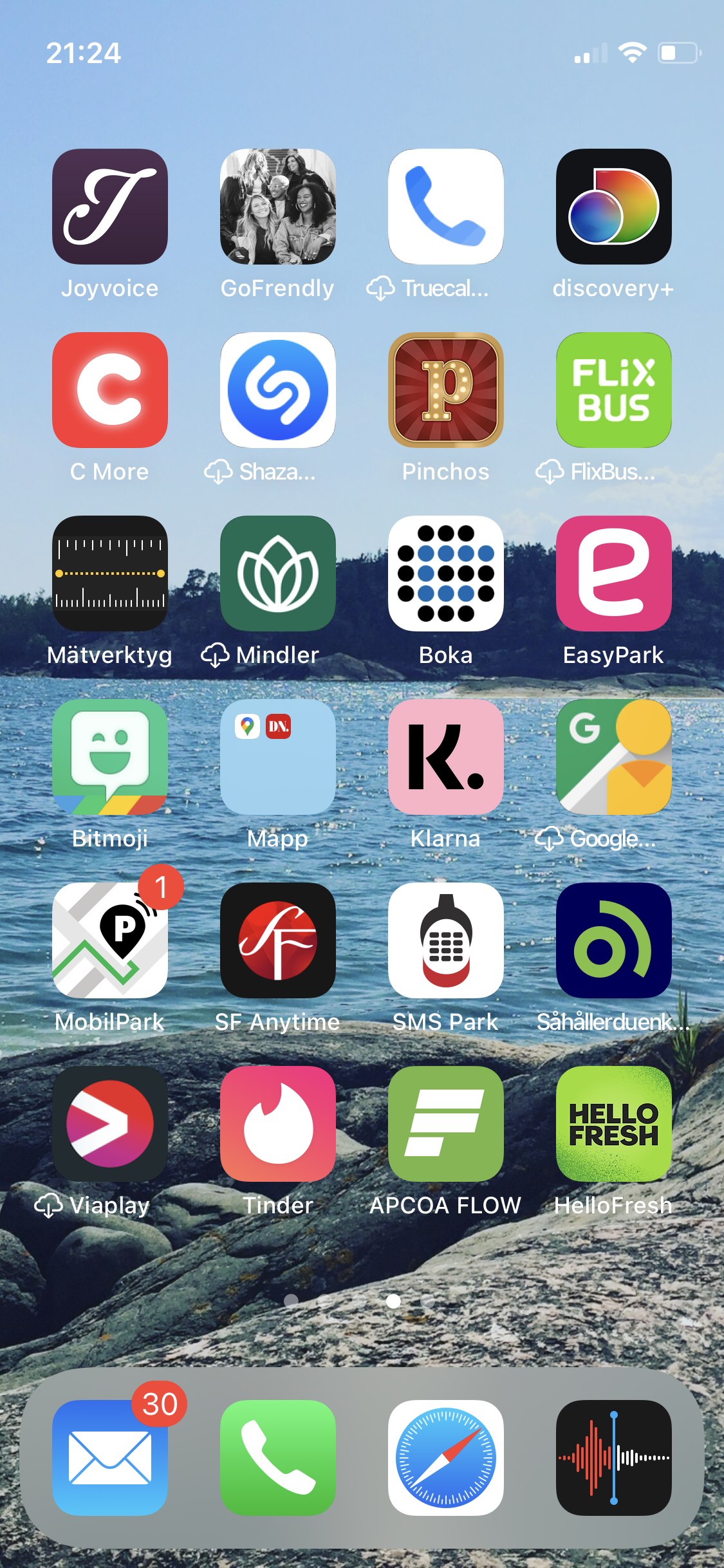The screenshot displays the home screen of an Apple mobile device organized into four app icons per row and seven rows in total. Here is a detailed breakdown of the apps:

1. **Top Row:**
   - Joy
   - Voice
   - Go Friendly
   - True Calc
   - Discovery Plus

2. **Second Row:**
   - See More
   - Shazam
   - Pin
   - Shows & Flicks Bus

3. **Third Row:**
   - Matchwork
   - TIG
   - Mindler
   - Bokeh
   - EasyPark

4. **Fourth Row:**
   - Bitmoji
   - Map
   - Klarna
   - Google Cloud

5. **Fifth Row:**
   - Mobile Park SF
   - Anytime
   - SMS Park
   - Schaller Donk

6. **Sixth Row:**
   - Viaplay
   - Tinder
   - App Coiflow
   - Hello Fresh

7. **Bottom Dock (Base Row):**
   - Email (showing 30 unread messages)
   - Messenger
   - Phone
   - Browser

Additionally, there is a red and white icon, though its details are not specified.

The neatly arranged rows display various applications for productivity, entertainment, and utilities, showcasing the device owner's diverse app usage.